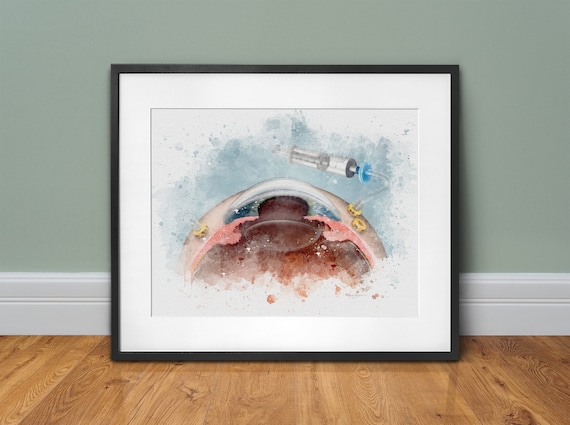The image features a framed abstract watercolor painting, leaning against a sage green wall with prominent white baseboards, set on caramel-colored wooden flooring. The black frame elegantly houses the artwork, accented by a white matting that creates a clean separation from its surroundings. The painting itself, marked by splotches of blue and hints of pink, centers around an ambiguous object that resembles an eyeball being held open by hands on either side. A syringe-like instrument is depicted protruding from this central object, connected to a yellow port. Accompanied by three distinctive circular yellow elements—two on the right and one on the left—the scene evokes a surreal, almost confusing atmosphere, emphasizing its abstract nature.